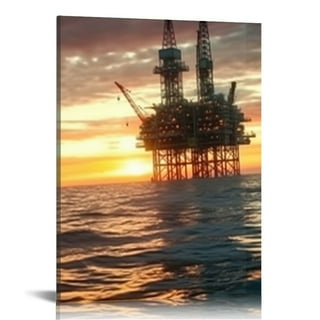The image is a highly detailed, clear, and colorful depiction of an oil rig set against a large body of water, likely at sunrise or sunset. The sun is positioned towards the left-center of the image, casting a bright, warm glow across the scene with hues of orange, yellow, black, gray, and off-white, while the cloudy sky adds depth to the background. The water below displays gentle ripples and waves with no white caps, indicating a relatively calm sea. The oil rig itself is prominently positioned in the top right of the image, consisting of two steel-supported towers with multiple working levels. Both the left and right sides of the rig feature crane apparatuses, adding to the industrial complexity of the structure. Though no boats, ships, text, or numbers are visible, the image's clarity suggests it was likely taken by a photographer from a nearby vantage point, possibly another boat. The overall scene captures the serene yet industrious atmosphere of the oil rig amidst the vast ocean backdrop.